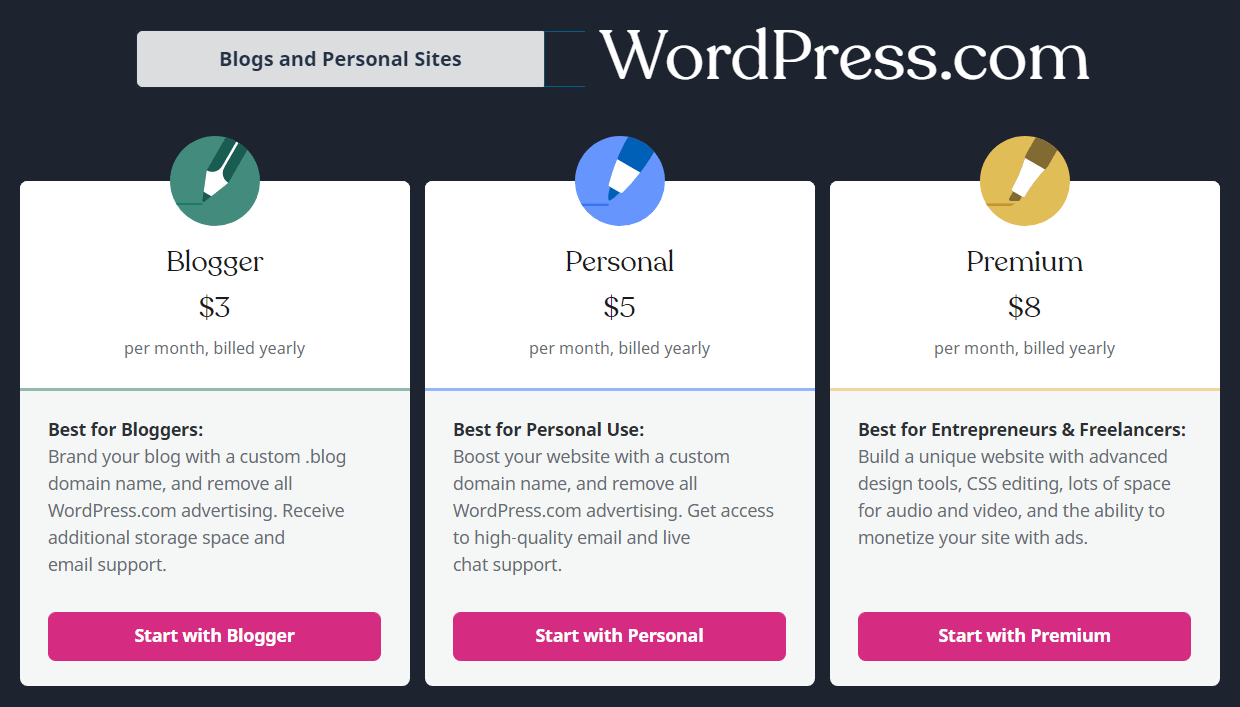The image is a screenshot from WordPress.com, detailing their Blogger, Personal, and Premium plans. At the top left corner, within a gray rectangle, it reads "Blogs and Personal Sites." Below, three options are presented in a horizontal layout:

1. **Blogger Plan**:
   - Represented by a green circle with a green pencil icon inside.
   - Priced at $3 per month, billed yearly.
   - Labeled as "Best for Bloggers."
   - Benefits include a custom .blog domain name, removal of WordPress.com advertising, additional storage space, and email support.
   - A pink button labeled "Start with Blogger" is available for selection.

2. **Personal Plan**:
   - Marked by a blue pencil icon.
   - Priced at $5 per month, billed yearly.
   - Labeled as "Best for Personal Use."
   - Similar calls-to-action include storage space benefits and email support.
   - A pink button labeled "Start with Personal" is provided for this plan.

3. **Premium Plan**:
   - Displayed with a yellow pencil icon.
   - Priced at $8 per month, billed yearly.
   - Aimed at users needing more advanced features.
   - Includes all functionalities meant to enhance the blogging experience.
   - A pink button labeled "Start with Premium" is also available.

Each plan is distinguished by a colored pencil icon and a detailed description of the offerings, along with a similarly styled call-to-action button at the bottom of each section.